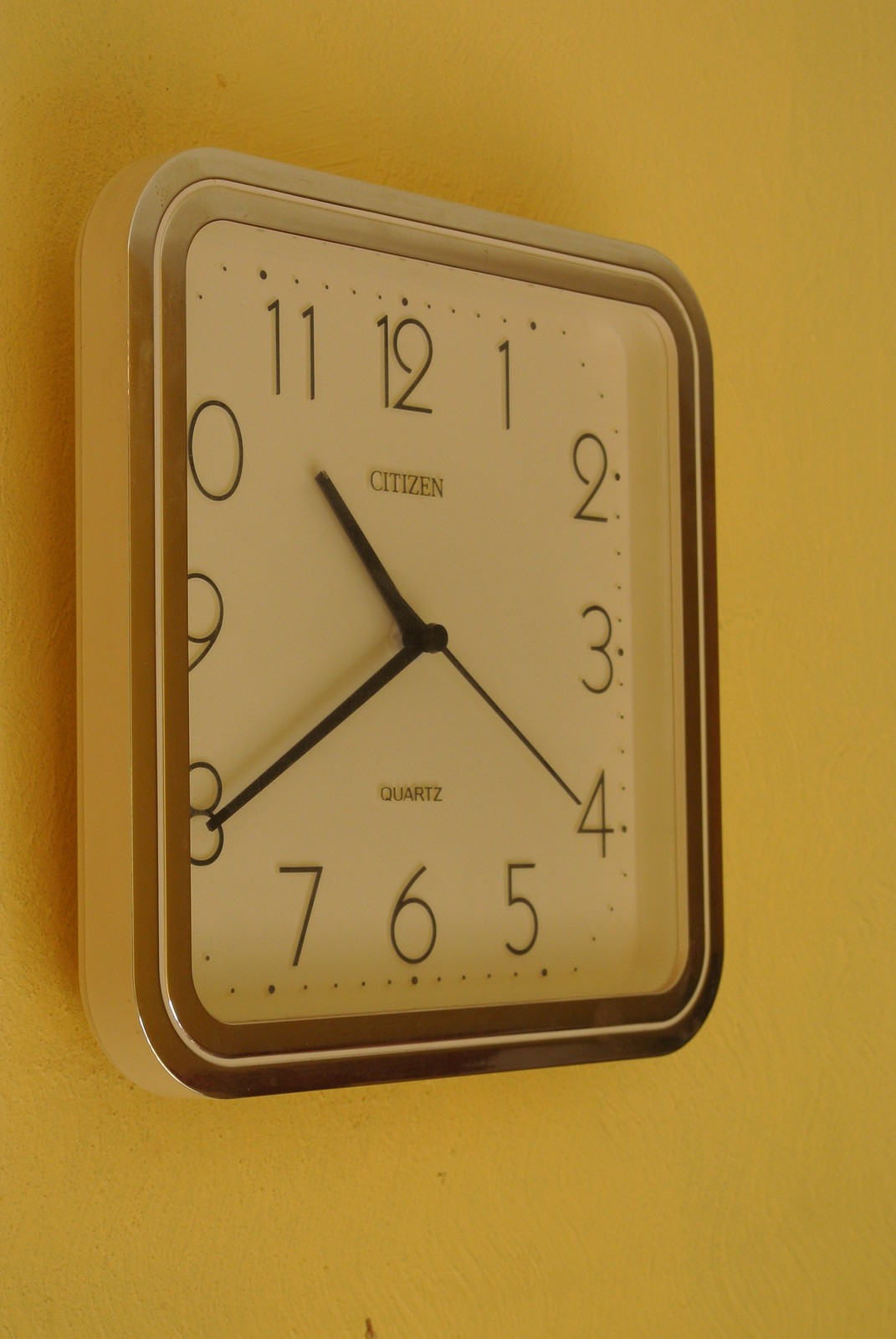This image features a prominently displayed analog clock mounted on a yellow stucco wall. The square clock, predominantly white with silver accents along its edges, occupies most of the frame. Detailed craftsmanship is evident in its design: a Citizen brand timepiece with a white face, flanked by alternating silver and white borders. The clock shows the precise time of 10:40 and 20 seconds, indicated by black hour, minute, and second hands. Each hour is marked with bold black numerals, and smaller black dots punctuate the spaces between the numbers, contributing to the clock's clean, minimalist aesthetic. At the bottom of the clock face, the label "quartz" is subtly printed, attesting to its timekeeping accuracy.